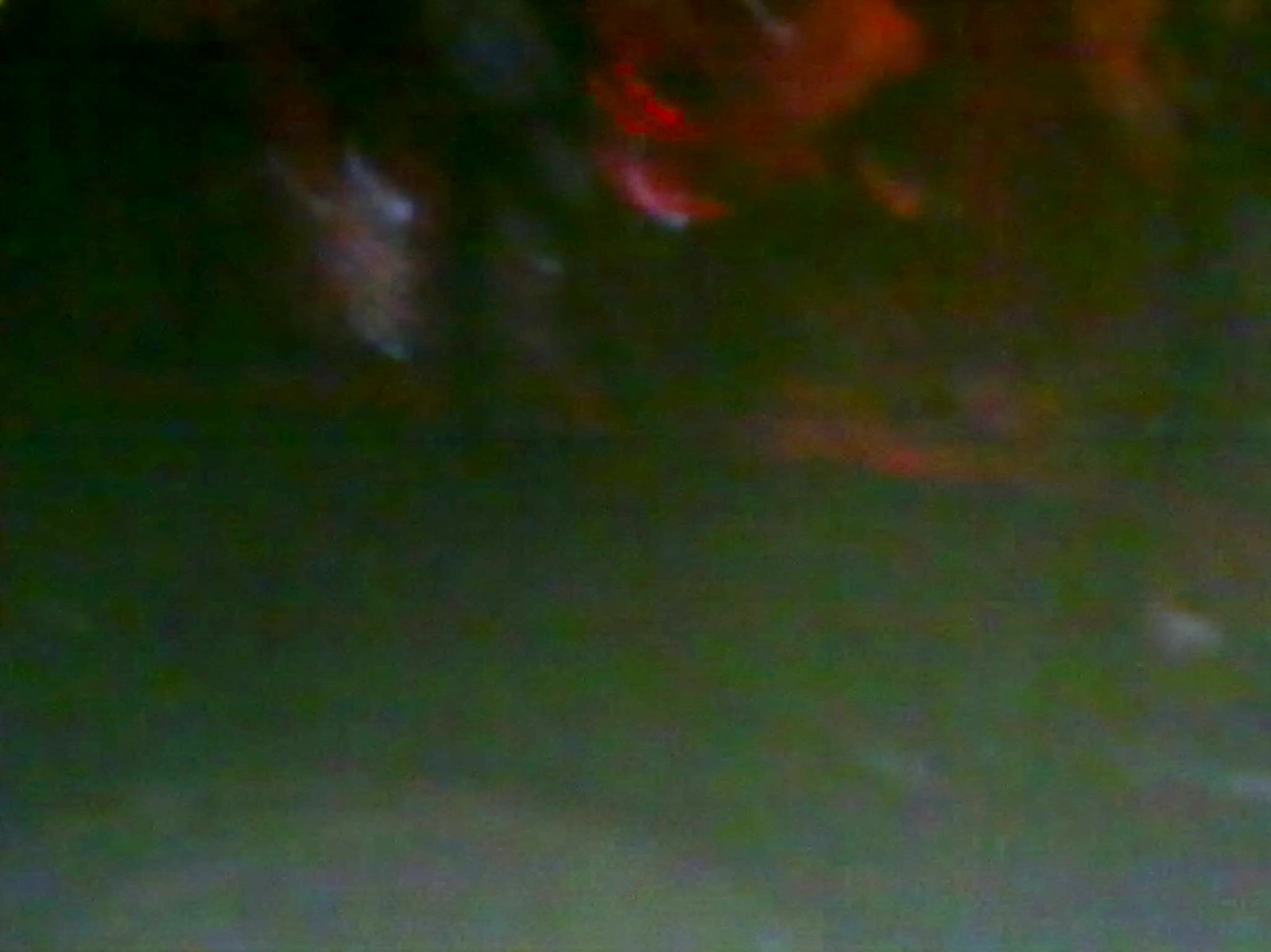This nighttime photograph, captured outdoors, is highly blurry and low in resolution, suggesting it may have been taken accidentally. Amidst the undefined forms, patches of green imply the presence of foliage or grass, hinting at an outdoor setting. The bright yellow hues likely originate from a flash, illuminating parts of the scene and contributing to its overall unclear quality. Additionally, sporadic reds might indicate the presence of a fire, a red light source, or some other unidentified object, while pervasive blacks accentuate the night’s darkness. The amalgamation of greens, yellows, reds, and blacks creates a chaotic, ambiguous image that leaves much to the imagination.